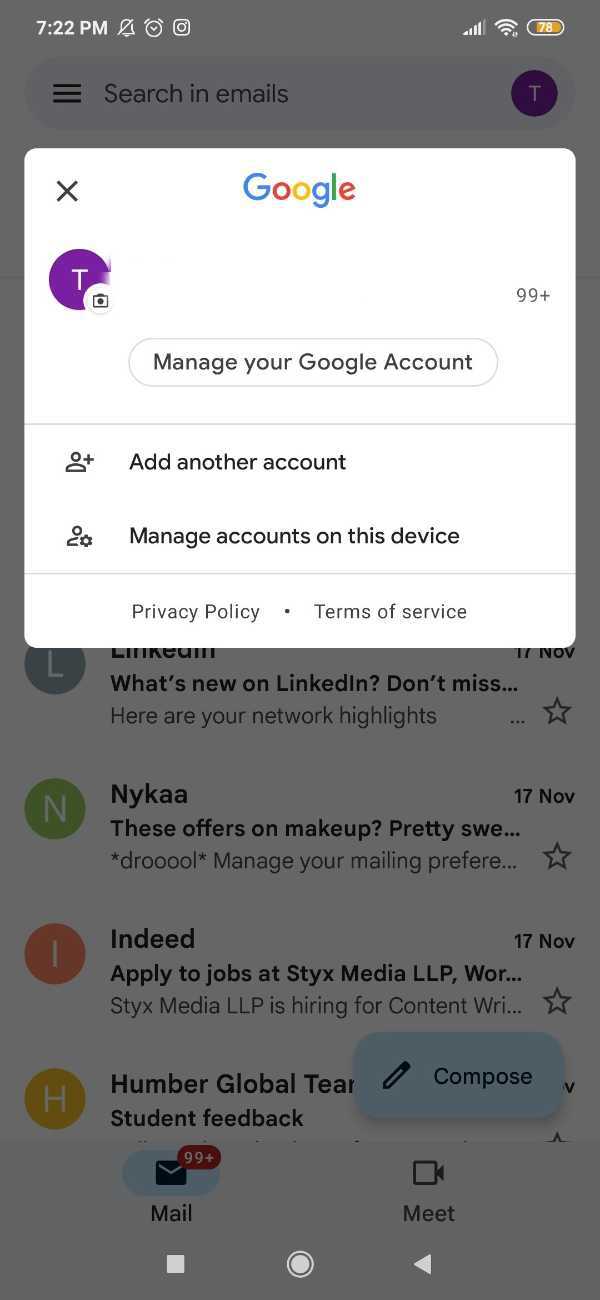A person is using their smartphone to check their emails at 7:22 p.m. Notifications are turned off, an alarm is set, and the battery is almost full. A pop-up from Google is currently displayed, obscuring part of the email screen. At the top, there's a "T" icon representing the user's account, a search bar for finding emails, and three lines indicating the settings menu. 

Visible emails include one from Nika about makeup offers dated November 17th and another from Indeed. The pop-up features a white box with a Google icon, the user's account logo (a purple circle with a white "T" and a camera icon for changing the profile picture), and options for managing the Google account. The two options provided are "Add another account" and "Manage accounts on this device," each accompanied by an icon of a person with a plus sign. At the bottom of the pop-up are hyperlinks to the "Privacy Policy" and "Terms of Service." In the grayed-out background, it’s visible that the user has 99 emails and an option to start a meeting via the "Meet" button with a camera icon.